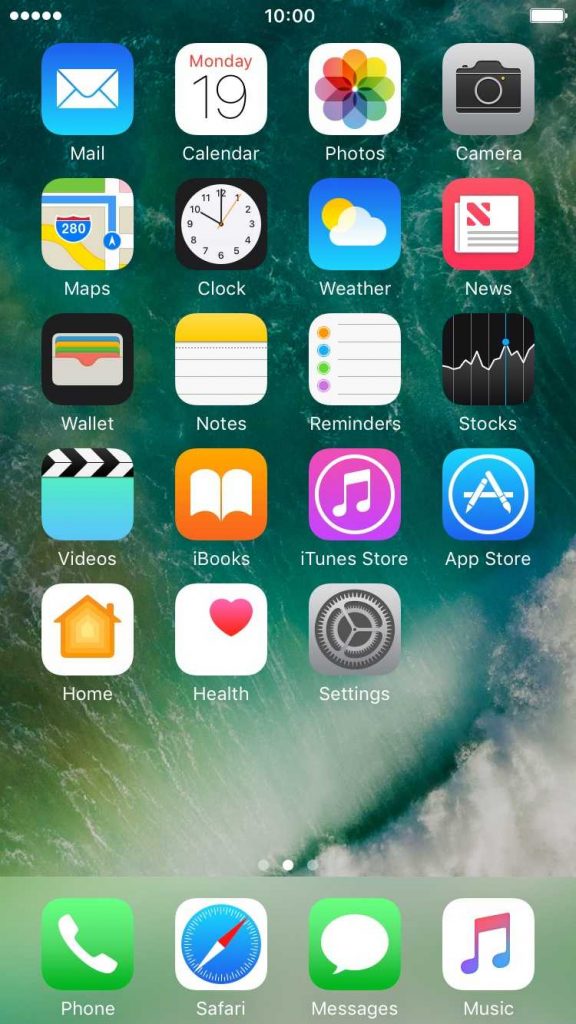This image showcases a smartphone home screen with a vivid and captivating ocean-themed background. Dominating the lower right corner of the wallpaper is a striking, frothy white wave rolling in from the sea. At the top center of the screen, the time is displayed prominently, reading exactly 10:00. Below the time, there is an organized grid of square-shaped app icons, featuring default applications such as Mail, Calendar, Photos, Camera, Maps, Clock, Weather, News, Wallet, Notes, Reminders, Stocks, Videos, iBooks, iTunes Store, App Store, Home, Health, and Settings.

Towards the bottom of the screen is a dock containing the user's primary apps, set against a greenish-gray bar. This dock includes icons for Phone, Safari (representing the internet browser), Messages, and Music. Each app icon is distinguishable by its unique color and design, such as the blue background of the Mail app and the clock graphic of the Clock app. Additionally, the upper right corner of the screen features a battery icon, indicating the smartphone’s current battery level. The neatly arranged icons and the scenic background provide a glimpse into the user's digital environment.